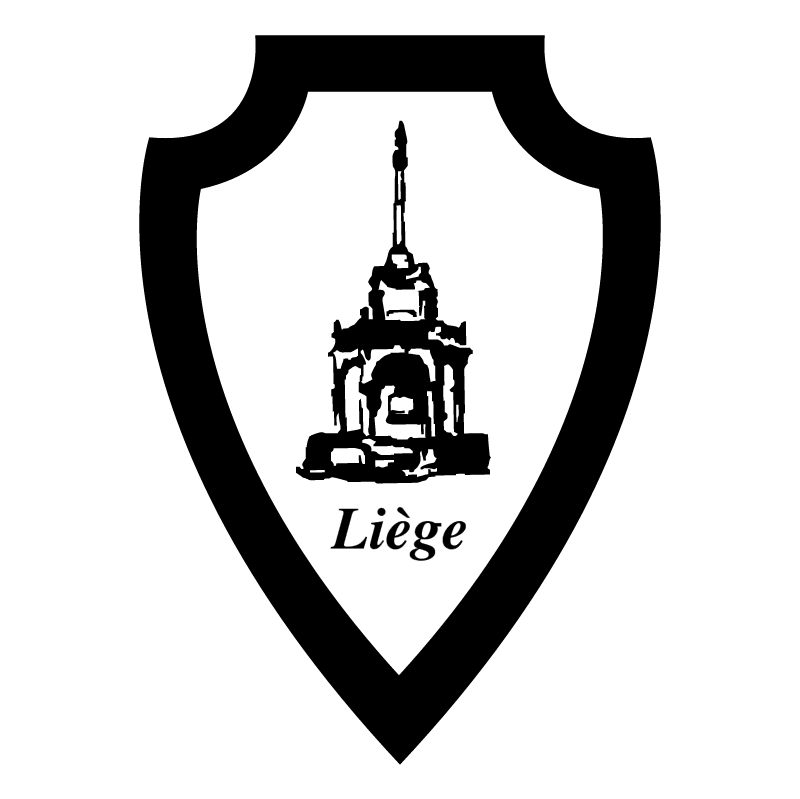The image showcases a minimalist, black-and-white emblem resembling a shield. The shield’s outer frame is black, while its center is white, creating a high-contrast design. In the middle of the shield is a black, hand-drawn illustration of a steepled building, possibly a church, featuring a thin rod or pole extending straight upward from the top. The structure suggests it might be a bell tower, with a hint of a bell visible inside. Below this architectural sketch, the text "Liège" is inscribed, with an accent mark over the "I," indicating the name of the Belgian city. The overall design of the emblem, with its downward-pointing arrow-like shape, gives it the appearance of a city symbol or logo for Liège.